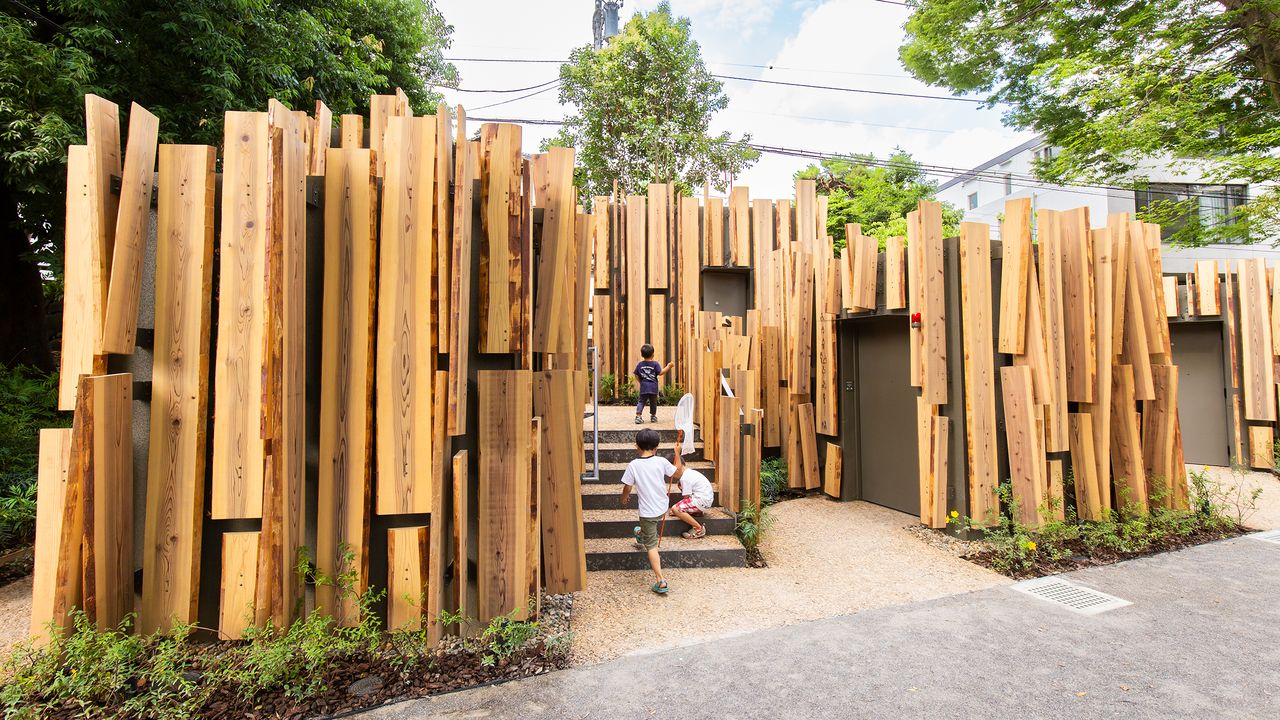The image captures a detailed scene of a park play area, centered around an artistic architectural structure known as the Tokyo Toilet, designed by Kengo Kuma. The structure is constructed from various polished, yet natural-looking vertical wooden planks in shades of brown and cream. It features multiple small buildings, each with dark brown doors set in matching frames. A staircase with six steps, covered in light gray gravel and concrete, leads to the structure. Three children are visible on the stairs, climbing up with their backs to the viewer. 

In the foreground, a dark gray street with light gray drainage grill runs diagonally from the bottom left to the middle right of the image. The ground beneath the children's feet appears to be a peach-colored soil. Some small plantings of greenery are visible next to the curb. In the background, on the top right, a multi-storied residential building is visible. The sky above is a light blue, adorned with light gray and white clouds. Power lines stretch across to a white building, adding to the urban landscape. Dark trees are also visible in the background, enhancing the outdoor setting of the photograph. The composition itself is a landscape orientation, capturing the overall natural and architectural elements of the scene with representational realism.